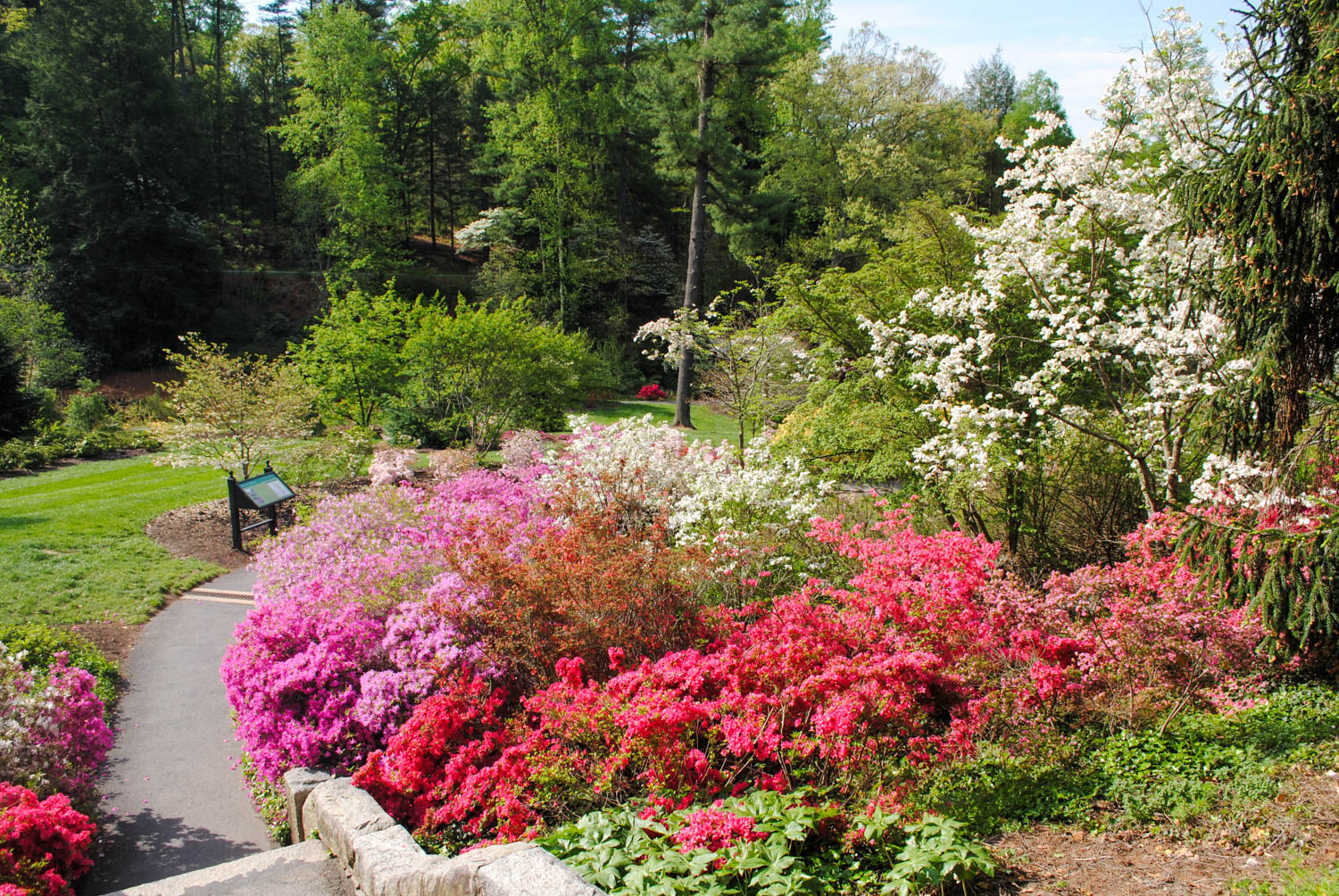This photograph captures a vibrant and picturesque park or possibly a botanical garden scene. Dominating the image are various trees and flowering plants in full bloom. The focal point is a winding sidewalk that begins with steps and then curves to the right, partially hidden by lush pink and white flower bushes. Alongside the pathway, meticulously arranged fuchsia pink, white, and red flowers create a vivid display, complemented by green shrubs and a well-maintained lawn to the left. Towering trees, including pine and oak, with their green foliage and splashes of white dogwood blossoms, create a rich, leafy canopy. In the background, a dense forest adds depth to the scene. A informational sign is prominently placed along the path, indicating points of interest in this scenic area. A small patch of blue sky is visible at the top, but the main focus remains the colorful, blooming flora that fills the image with natural beauty.